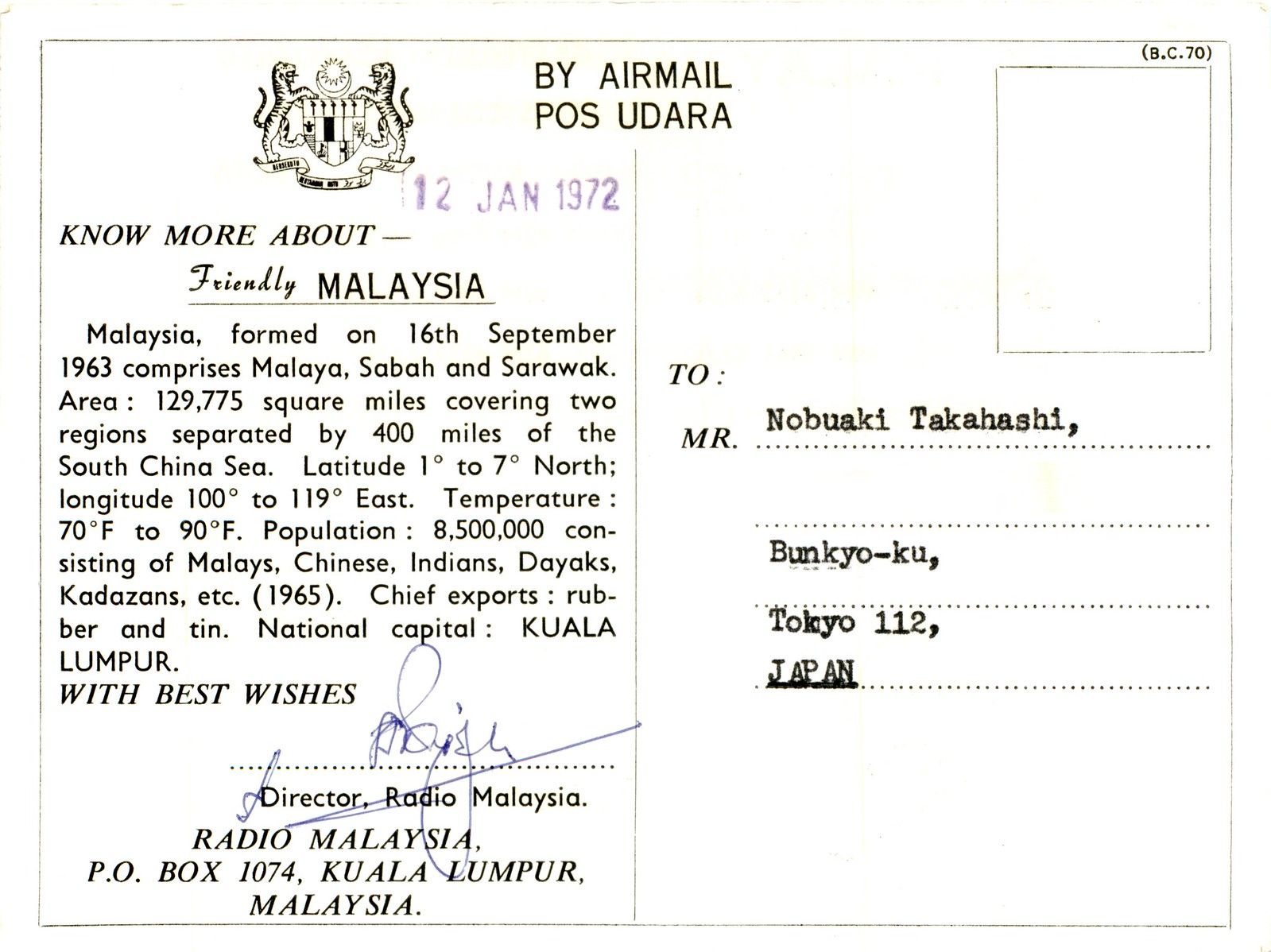The image showcases the back side of a white postcard divided by a faint vertical line down the middle. On the left side, there is a heraldic crest featuring tigers and a sun, next to text that reads "Know More About Friendly Malaysia." Below this, a paragraph provides information about Malaysia's formation on September 16, 1963, detailing that it comprises Malaya, Sabah, and Sarawak, covering 129,000 square miles across two regions separated by 400 miles of the South China Sea. Beneath the paragraph, the text concludes with "With Best Wishes, Director Radio Malaysia," followed by a signature. Additionally, there is a purple stamp dated "12 Jan 1972." On the right side, the upper section has a designated space for a stamp. Below it, the text "To: Mr. Nobuaki Takahashi" is typed, with the address "Bunkyo-ku, Tokyo 112, Japan" neatly printed underneath. The top center prominently features the text "By Air Mail," with "POSE UDARA" inscribed below it in large letters.